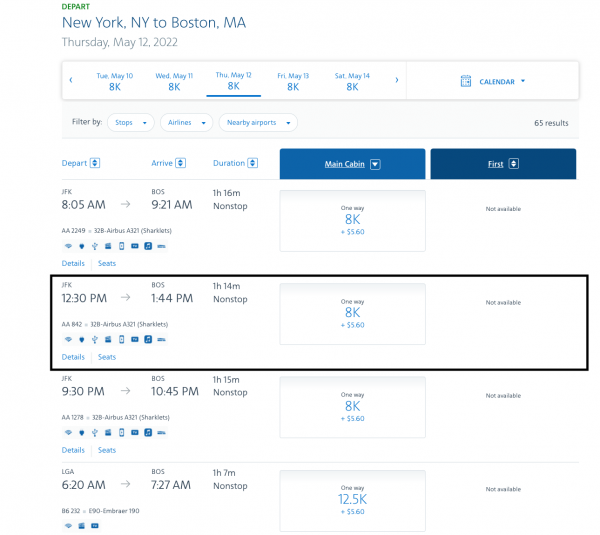Set against a crisp white background, the image displays a detailed travel itinerary in various text colors for clarity. In the upper left corner, small green text reads "Depart," followed by blue text indicating the journey from "New York, New York to Boston, Massachusetts." Directly below, gray text specifies the date, "Thursday, May 12, 2022." 

In prominent blue text, dates are listed sequentially as "Tuesday, May 10," "Wednesday, May 11," "Thursday, May 12," "Friday, May 13," and "Saturday, May 14." The date "Thursday" is underlined in blue to highlight its importance.

Beneath these dates, an outlined black box details a specific flight option: departing from JFK Airport at 12:30 PM, arriving in Boston at 1:44 PM, with a flight duration of 1 hour and 14 minutes. The flight is one-way and listed as costing "8K plus 560."

To the right of this box, there's a smaller box labeled "Not Available."

Further below, another flight option is displayed in a similar format: departing from JFK at 9:30 PM and arriving in Boston at 10:45 PM, with a duration of 1 hour and 15 minutes. This flight is also one-way, priced at "8K plus 560" in blue text.